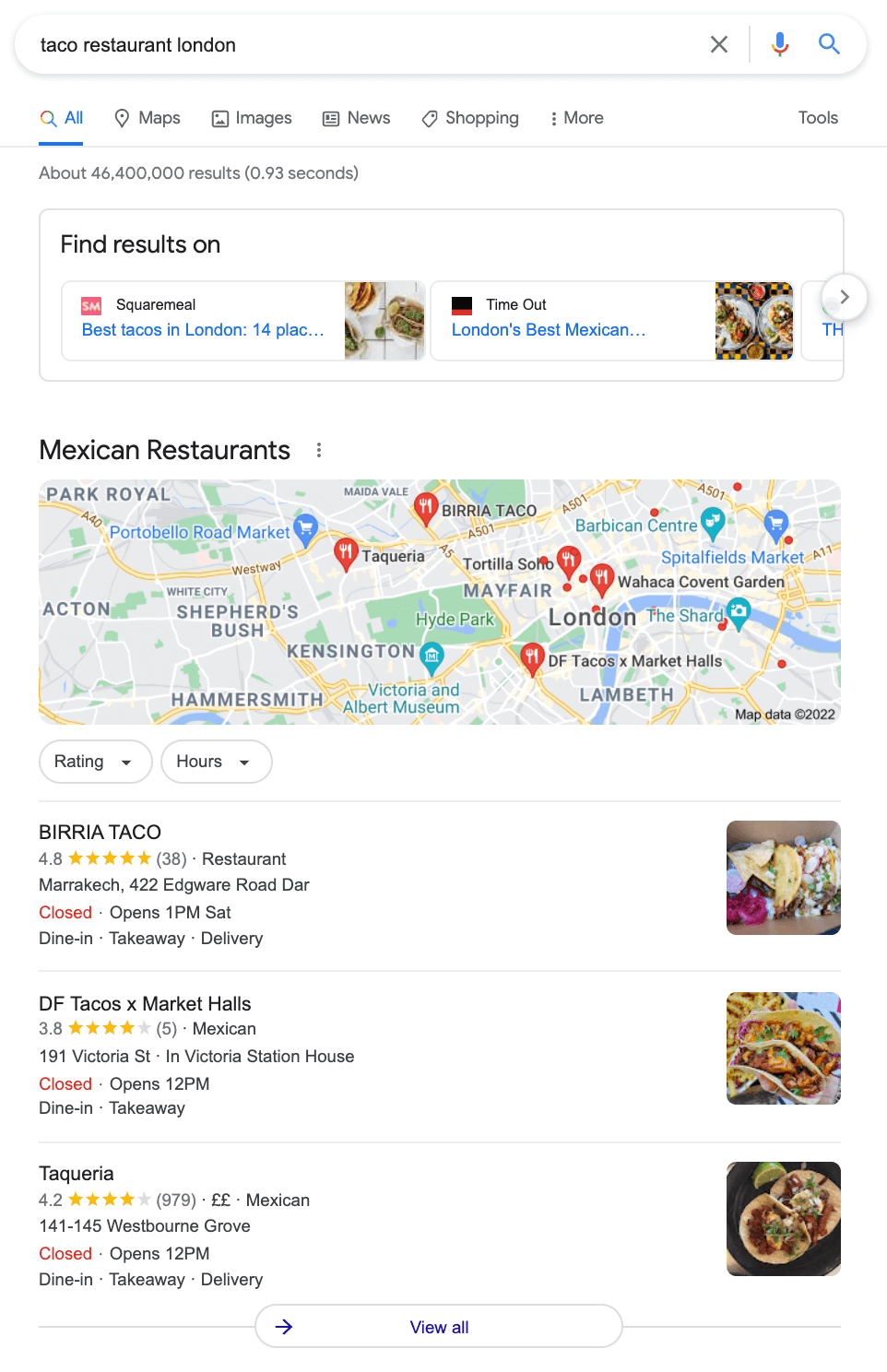The image depicts a screenshot of a website where a user is searching for taco restaurants in London. The website features a predominantly white background. At the top of the page, the user has entered "taco restaurant London" into the search bar. Instead of selecting options like Maps, Images, News, Shopping, or Tools, they have chosen the "All" category. The search results indicate approximately 46,400,000 results found in 93 seconds.

Below the search bar, there's an advertisement section promoting services like Square Meal and Time Out. Underneath the ad, a map of the London area is displayed, labeled with "Mexican restaurants." The map is marked with five red pins, highlighting various taco restaurant locations in the city.

The restaurants listed include:
1. **Birria Taco**
2. **DF Tacos and Market Falls**
3. **Taqueria**

Each restaurant listing features enticing images of the food, showcasing the dishes in high detail, which look incredibly appetizing. At the bottom of the listings, there is a white box with purple text that provides an option to "View More."